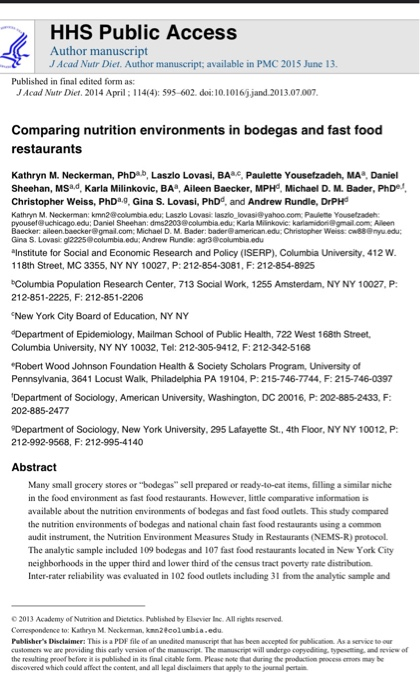This image depicts a website with a clean, white background. At the top, there is a thin black line followed by a white section, beneath which lies a gray banner. The banner reads "HHS Public Access" with "HHS" and the initials "P" and "A" in "Public" and "Access" capitalized. Below this, the text indicates "Author Manuscript" and "Published in Final Edited Form." 

The main title of the content is "Comparing Nutrition Environments in Bodegas and Fast Food Restaurants." Following the title, the document lists the participants who contributed to the writing, their respective goals, and the involved research centers. The section titled "Abstract," marked in bold black text, begins by explaining that many small grocery stores, referred to as "Bodegas," stock self-prepared and ready-to-eat items, serving a similar niche in the food environment as fast food restaurants. Despite this, there is limited comparative information available about the nutrition environments of Bodegas versus fast food outlets. 

The study mentioned in the abstract aimed to compare the nutrition environments of Bodegas and national chain fast food restaurants using a standardized audit tool from the Nutritional Environment Measure Study in restaurants. At the bottom of the image, there is a note indicating that the article was published in 2013 by the Academy of Nutrition and Dietetics and is available through Elsevier, Inc.